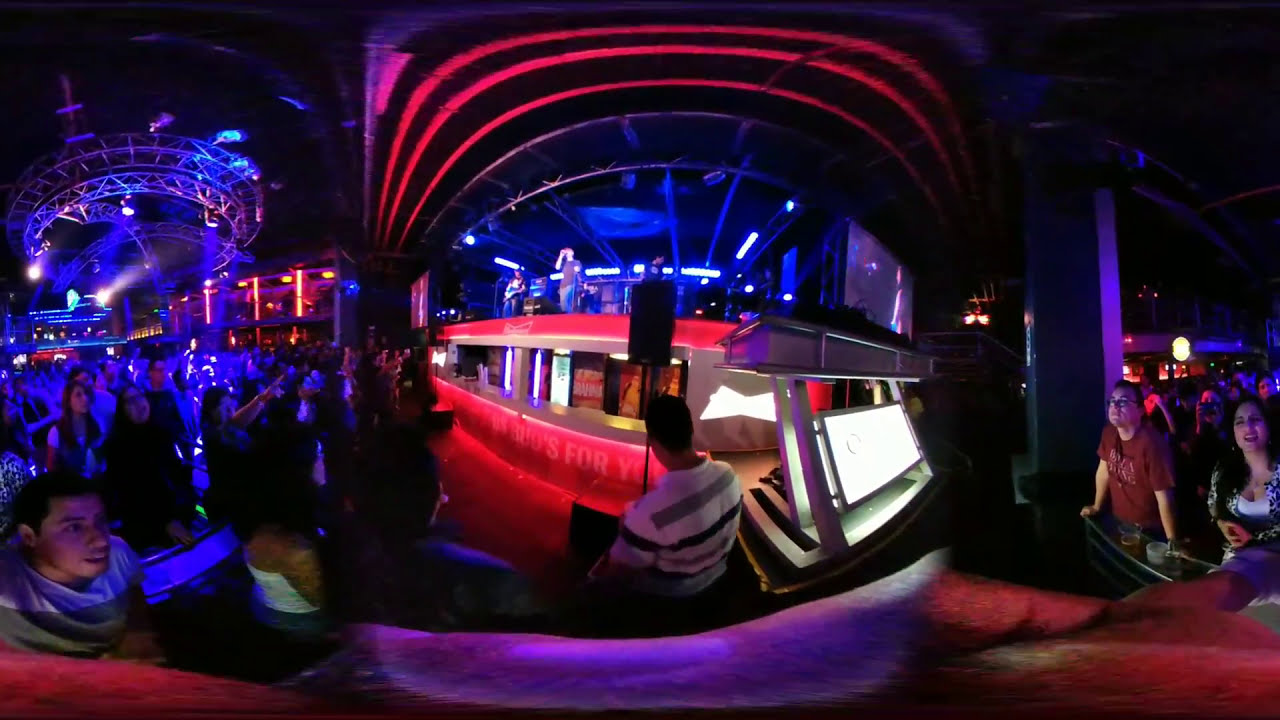The image captures a vibrant event set in an indoor venue designed to mimic an outdoor atmosphere. The central focus is a large, brightly lit stage, adorned with blue and red lights, creating a visually dynamic scene. The stage, which features multiple performers including one with a microphone and another with a guitar, appears to be divided into a main stage and a secondary area, possibly for an orchestra. Surrounding the stage is a crowd of onlookers, some of whom appear to be enjoying drinks. Notable figures in the audience include a man wearing a red shirt and glasses, and another person in a striped white, gray, and black shirt. At the forefront, there is a striking red, boat-like structure with curving ridges, which adds a unique architectural element to the setting. The various lights create a dramatic ambiance that enhances the overall visual appeal of the scene.